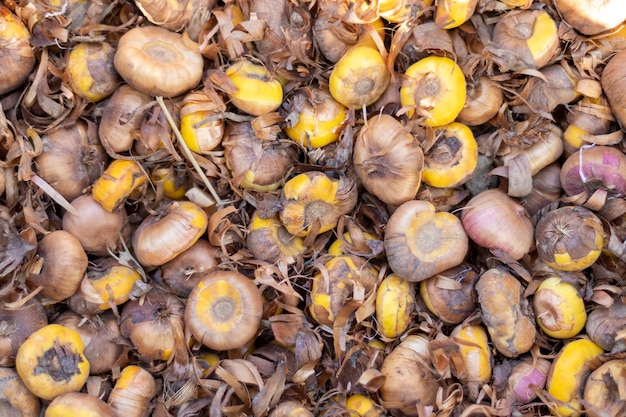The image depicts a large bushel, likely around a hundred bulbs, with each bulb showcasing a vibrant yellow hue. These bulbs, though resembling onions with their papery brown, maroon, and purple-tinged skins, are not onions. Some may mistake them for tulip bulbs or other plant bulbs ready for planting, contrasting with the pointed ends indicating their top and root. The scene suggests a farmer's market setting, characterized by the chaotic arrangement and peeling skins scattered among the bulbs. The bulbs vary in their states of freshness, with some appearing fully yellow and others showing signs of drying out. This visual complexity evokes a sense of abundance, and the mixture of loose skin adds to the rustic and ready-to-plant impression of the whole bushel.